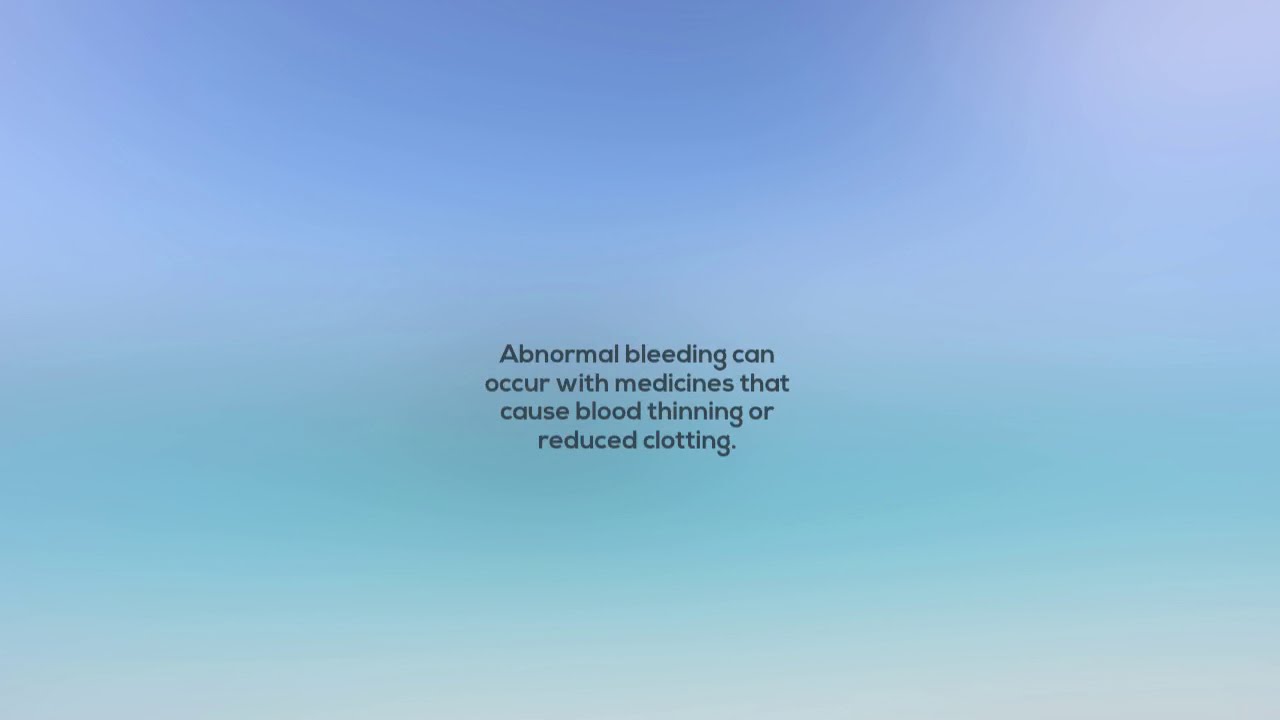This image features a large, multicolored rectangle with a gradient-shaded background transitioning from blue at the top to gray in the middle, then to green, and back to gray at the bottom. The center of the image prominently displays a small section of text reading, "Abnormal bleeding can occur with medicines that cause blood thinning or reduced clotting." The background surrounding the colored box consists of various shades of blue, ranging from lighter blue to teal, creating a blurred, simple backdrop. The text is centrally positioned within the colored rectangle and is the only content visible in the image, suggesting it is likely an informative medical slide or part of a presentation regarding medication side effects.